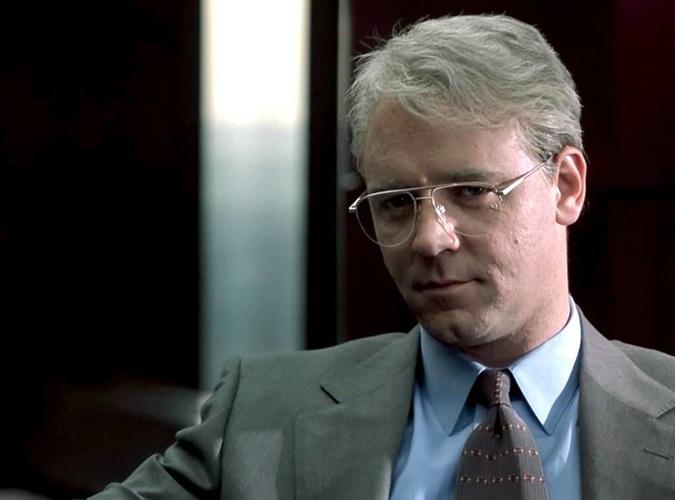This photograph, possibly a frame from the film "The Insider," features an older white man, identified as Russell Crowe. He has short, graying hair brushed back and wears clear, light gold-rimmed glasses. His attire includes a solid light blue shirt paired with a medium gray suit jacket. Completing the ensemble is a dark gray tie, adorned with brown horizontal stripes and rows of small white dots. Crowe has a serious expression, looking slightly past the camera with a cunning gaze. The background is predominantly dark, with a white stripe running vertically on the left side, possibly suggesting an elevator interior.